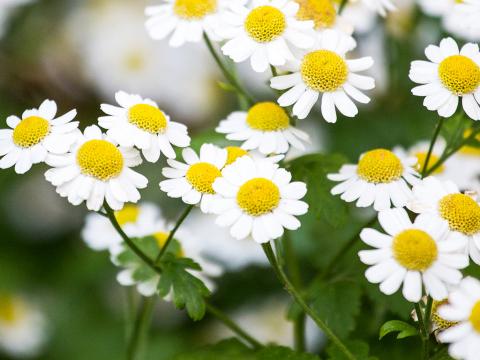This vibrant and detailed photograph captures a close-up of numerous white-petaled daisies with bright yellow centers, highlighted against a backdrop of lush green leaves and stems. The image, taken during the daytime, showcases an array of over a dozen daisies that dominate the scene, creating a lively and prolific display suggestive of a well-pollinated and thriving garden. The background gradually fades into a blur, drawing the viewer’s focus to the crisp, vivid details of the daisies in the foreground. The overall composition spans primarily from the center to the right side of the image, with a few petals extending off the left edge. The colors are striking, featuring intense yellows, whites, and greens, which contribute to the photograph's cheerful and vibrant atmosphere.